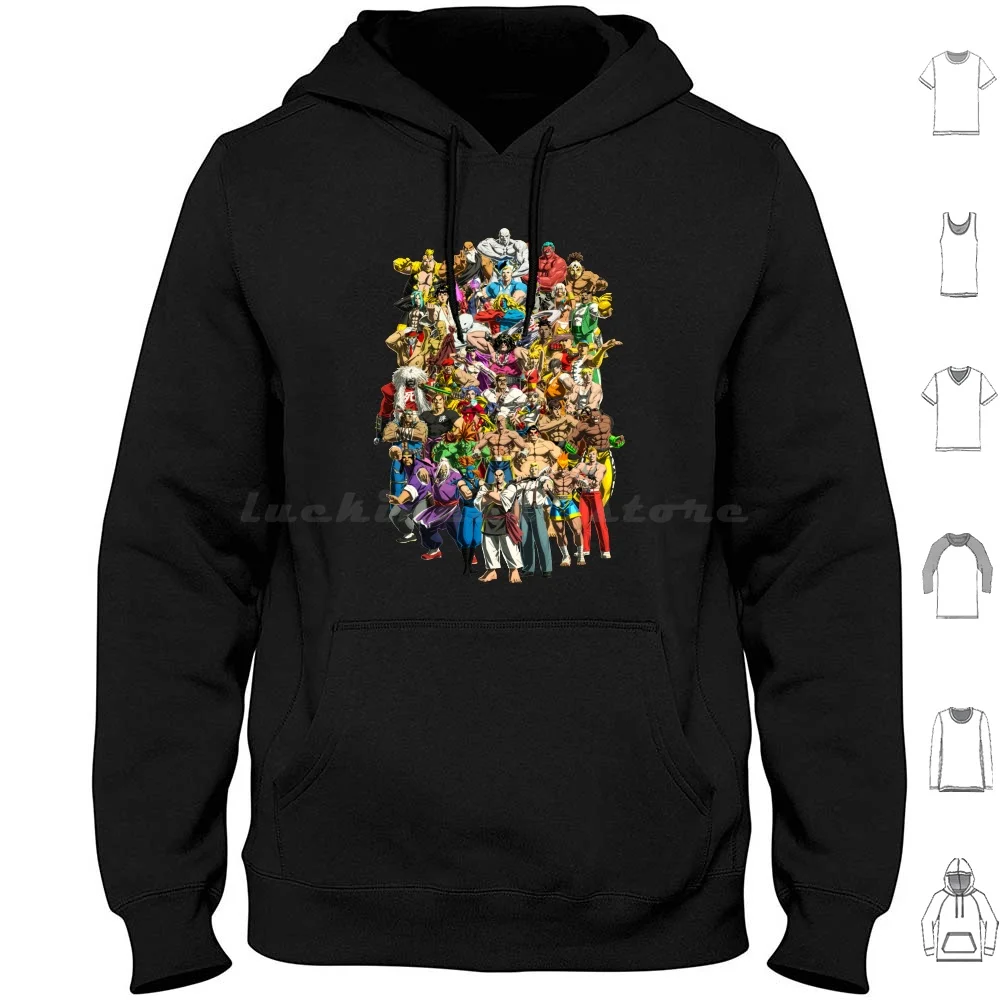The image showcases a black hoodie prominently displayed against a white background, designed for a catalog layout, likely intended for a website. The centerpiece of the hoodie features a vivid, colorful graphic comprising dozens of animated characters, including superheroes and cartoon martial artists. The characters, depicted in a variety of colors such as yellow, black, brown, purple, red, blue, green, teal, and orange, are all grouped together in dynamic poses, facing the viewer. This intricate design is centrally placed on the front of the hoodie. To the right of the main hoodie image, there are six black and white line drawings illustrating different shirt styles available, including short sleeve, tank top, v-neck, baseball tee, long sleeve tee, and hoodie. These drawings serve as a reference for how the same design might appear on other apparel styles. The layout is minimalist, ensuring that the black hoodie and its detailed graphic remain the focal points of the page.